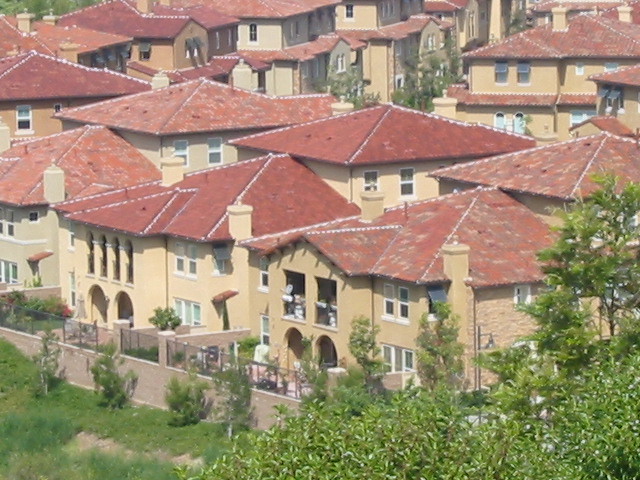This image showcases a picturesque gated community reminiscent of European architectural styles, possibly located in Southern California. The two-story homes, unusual for a region known for its single-story ranch-style houses, feature distinctive arches on the ground level and are indicative of high-end properties, likely valued at over a million dollars. In the foreground, a gate marks the entrance to this exclusive neighborhood, hinting at its private and secure nature.

The homes are substantial in size, suggesting luxury and spacious living areas. In the background, there are additional archways that might lead to backyard areas, adding to the elegance of the property design. The scenery is complemented by lush foliage, hinting at a location near the mouth of a canyon, which adds a natural and serene backdrop to the setting. A street is visible in the upper right corner of the image, further defining the layout of this well-planned community.